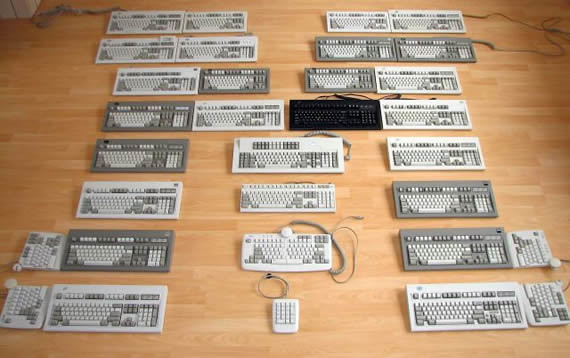This image, taken from about human eye level, shows a collection of computer keyboards meticulously arranged on a light brown wooden floor. The keyboards, primarily white with some gray and a single black one, form a large capital "M" pattern. The layout includes several keyboards turned sideways and a few smaller keypads, with a distinctive white touch keypad positioned at the bottom point of the "M." Despite many having visible cords, most keyboards do not show cables. The scene is photographed at an angle of approximately 40 degrees, highlighting the creative arrangement of the keyboards on the floor.